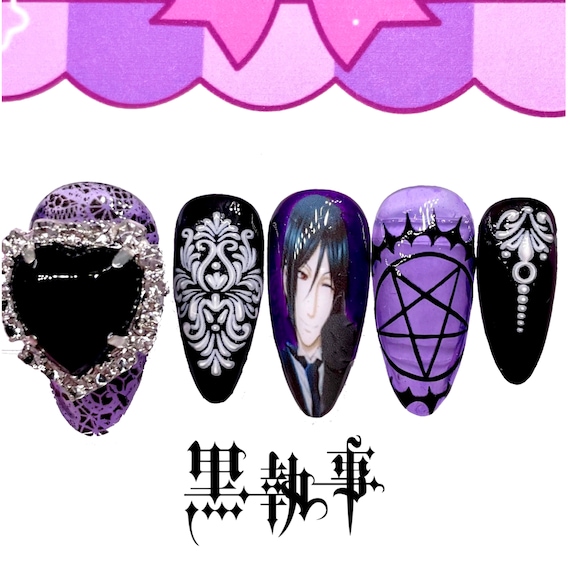The image showcases a set of five elaborately decorated fingernails, each with its unique design and intricate details, predominantly in purple, black, and white hues. The leftmost nail features a black background accentuated by delicate purple lace webbing, though this is mostly obscured by a prominent black heart-shaped jewel encrusted with smaller silver or clear gemstones around it. The second nail boasts a symmetrical white floral motif over a black background, reminiscent of an ornate fleur-de-lis. The third nail depicts an anime character's face on a dark purple backdrop, showing the character in a collared shirt, dark tie, and headband although the image is slightly distorted due to the nail's narrow shape. The fourth nail is medium purple, almost lavender, decorated with an inverted pentagram encircled by spiky diamond shapes, evocative of round teeth when viewed through the negative space. The rightmost nail, set against a dark background, features a white design with a fleur-de-lis shape at the top followed by a circle and a line of descending dots. The overall scene is framed by what appears to be a purple and pink scalloped awning at the top and gothic-styled Asian characters at the bottom.